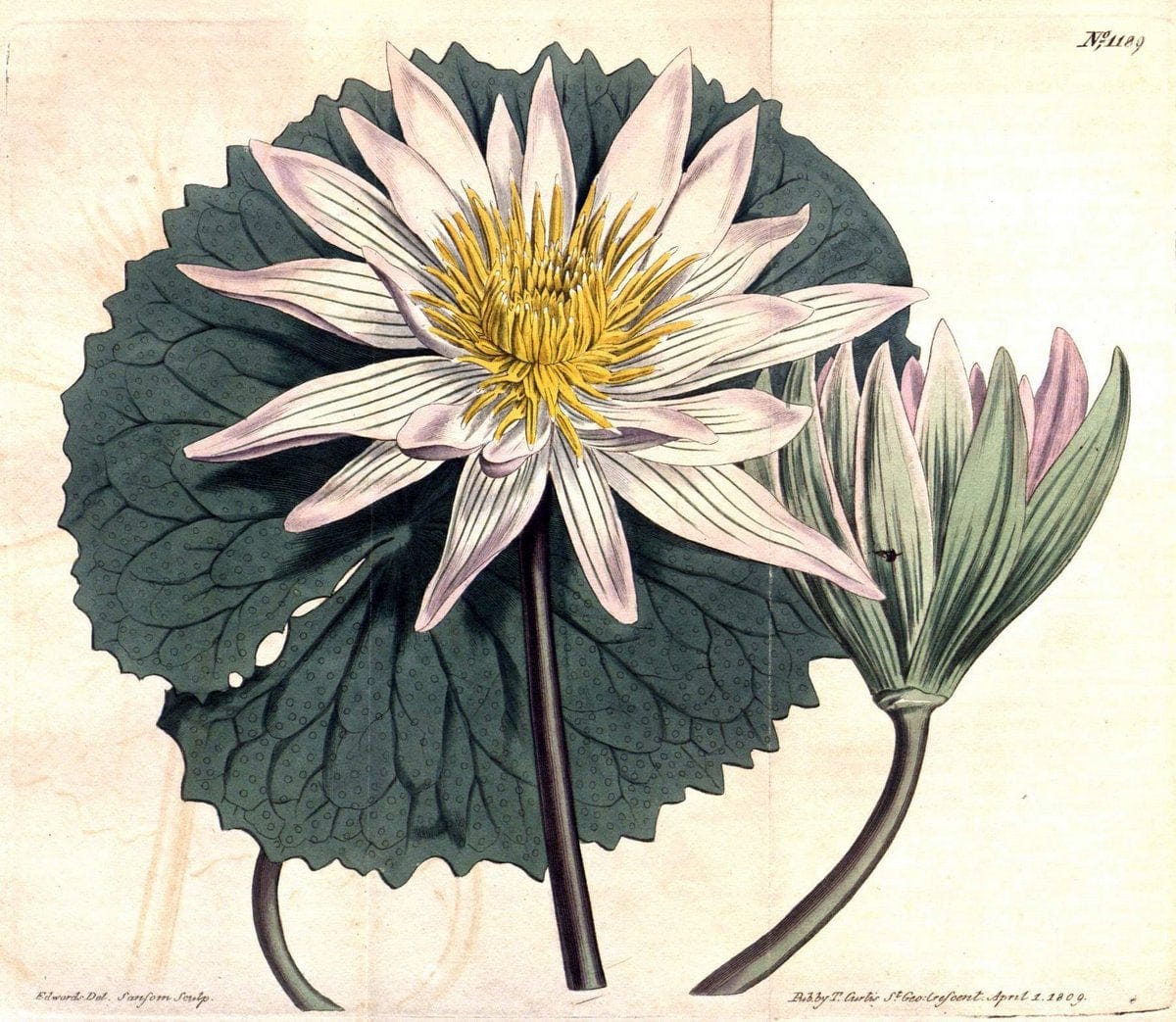This detailed painting, likely resembling an old botanical illustration from the late 19th or early 20th century, beautifully captures a meticulously rendered water lily on a slightly off-white sheet of paper. The sheet appears to be slightly aged, with a single fold running through it and scattered tiny brown dots adding to its antique appearance. The background hints at light brown and white color variations, enhancing the vintage effect.

In the upper right corner of the paper, the marking "N118G" is visible, possibly an identification number for the plant. Below this marking, some indistinct cursive handwriting, which seems to be a date—possibly "April 2nd, 1879" or a similar year—is faintly visible, adding a historical touch to the illustration.

The water lily itself is striking, featuring a prominent open blossom at the center with 23 long, pointed petals that radiate like sun rays. Each petal is predominantly white with subtle hints of pink, especially near the base, and demonstrates delicate vein details. The vibrant yellow center of the flower is composed of fine, hair-like pistils and stamens that resemble a miniature dandelion clock.

Accompanying the blooming flower is an unopened bud, positioned to the lower right. This bud reveals green hues on its exterior with subtle touches of pink and white as it begins to open. Both flowers are anchored by stems emerging from a large, round lily pad located in the background. This pad features scalloped edges and dark green veins with lighter green spots dispersed throughout. It has a split at the top, giving it a heart-like shape, enhancing the botanical accuracy of the depiction.

Various indistinct cursive letters adorn the bottom left and right corners of the paper, possibly written in fancy calligraphy, though they remain illegible. Overall, this art piece, potentially part of a flower book or plant portfolio, meticulously presents the water lily in exquisite detail, combining botanical precision with artistic elegance.